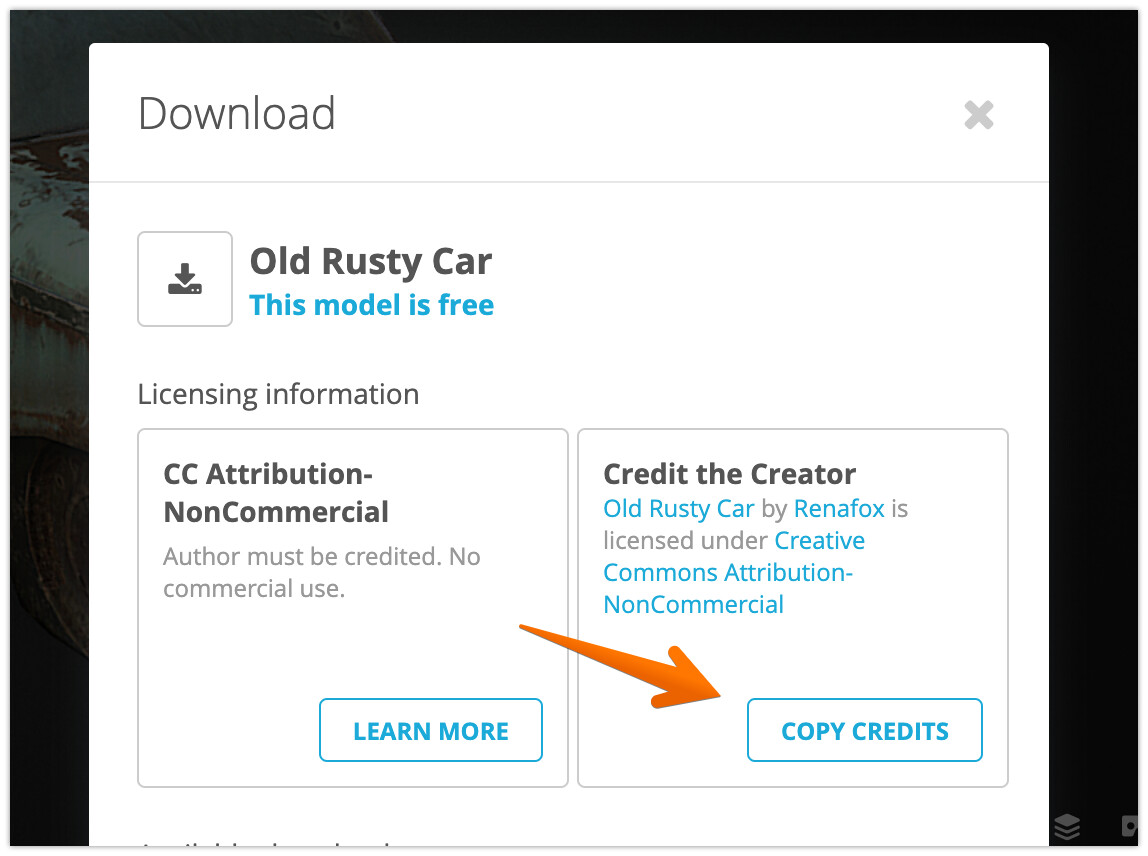This image appears to be a screenshot of a web page. The layout is in a landscape orientation, with a dark gray background. On the left-hand side, there is a slightly visible, rust-colored object in the background. While difficult to ascertain its precise nature, it resembles a rusted vehicle, featuring shades of brown with patches that appear dark white, indicative of its aged and corroded state.

At the center of the image is a large white rectangle, prominently displaying the following elements:
- At the top of this rectangle, "Download" is written in bold black text.
- Positioned on the right-hand side, there is an 'X' icon, typically suggesting a close button.
- A horizontal line separates the header from the section below it.
- Below the line, the text "Old Rusty Car" is written in black.
- Underneath the title, in blue text, it states, "This Model is Free."
- To the left of this message is a download button.

Further down, the text "Licensing Information" is displayed, followed by two rectangular boxes at the bottom:
- The first rectangle reads "CC Attribution, Non-Commercial."
- The second one states "Credit the Creator."

Overall, this detailed layout suggests a downloadable model of an old rusty car being offered for free, with clear instructions on licensing and attribution requirements for the user.